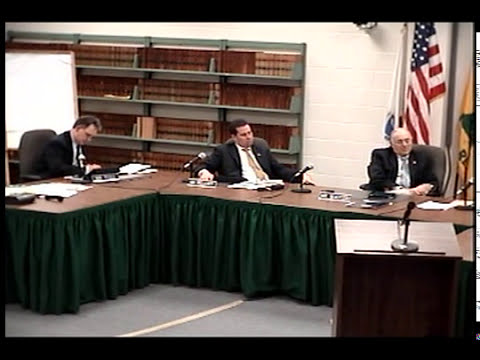This image depicts a formal meeting setting, possibly a government or municipal gathering from the late 90s or early 2000s. The scene centers around three Caucasian men with dark hair wearing dark suits and white dress shirts, each equipped with a microphone. They are seated at an L-shaped table draped in an outdated, frilly dark green skirt. The table appears to be composed of brown folding sections, covered with papers and possibly other office tools. To the right of the men, there is a wood podium with a microphone mounted on it. 

In the background, an older man stands near an American flag beside an old steel bookcase filled with brown encyclopedias. The room’s floor is covered with white or gray carpet, and the walls are painted white. The men at the table are engaged in different activities: one is writing or working on a computer, another, wearing a gold tie, gazes into the distance, and the third is seated, looking towards the right as if listening to someone off-frame. The image is framed with black rectangles at the top and bottom, suggesting it could be a screen capture or a photograph from a broadcast or a document from that era.